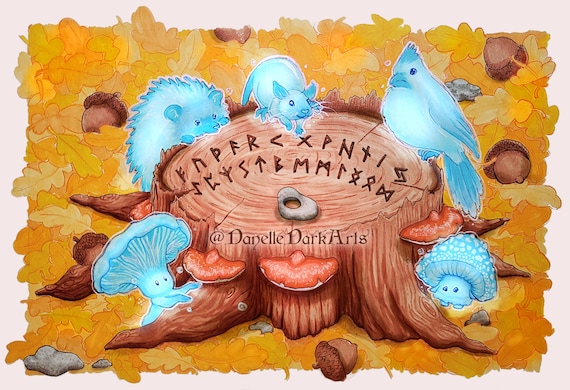The image is a detailed, rectangular artwork that features an artist's rendering of a tree stump at its center. The tree stump, which appears to be cut off at the bottom, is drawn in various shades of brown with mushrooms sprouting from its sides. Surrounding the stump are bright blue mythical creatures, including figures that resemble a bird, a mouse or rat, a hedgehog, and two mushroom people, giving the scene a mystical touch. Script in a runic or secret language crosses the middle of the image, with the text "at Danielle Dark Arts" inscribed in black. The background is a rich tapestry of golden leaves, evoking an autumnal feel, interspersed with acorns and small, indeterminate gray objects. The entire composition is framed by a subtle white outline.